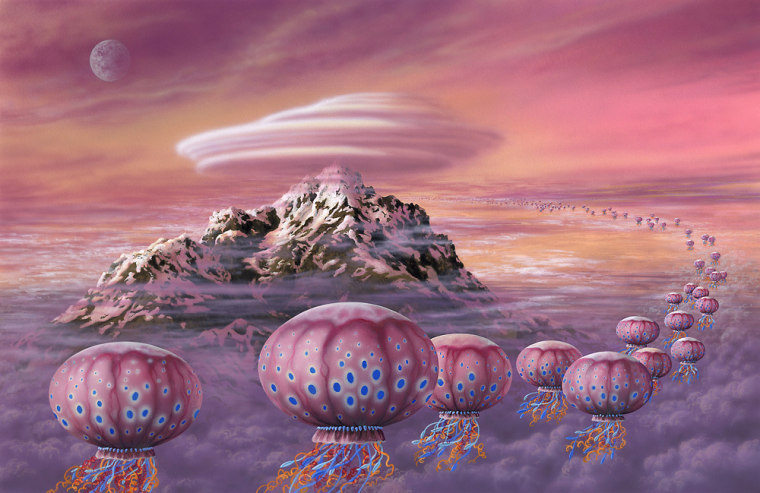In this fantastical image, an enchanting scene unfolds with round squid adorned with confetti-like tentacles floating in pairs, extending endlessly behind a snow-capped mountain peak that juts majestically from a sea of clouds. The sky is a dreamy blend of pink and purple hues, adding to the surreal atmosphere. A spaceship-shaped, thick white cloud hovers above the peak, enhancing the otherworldly essence of the picture. In the top left corner, a glowing full moon peeks out, casting its soft light across the scene. The squid, reminiscent of whimsical hot air balloons, boast vibrant streamers in shades of yellow, gold, red, and blue, creating a kaleidoscope of colors against the fluffy pink clouds below.